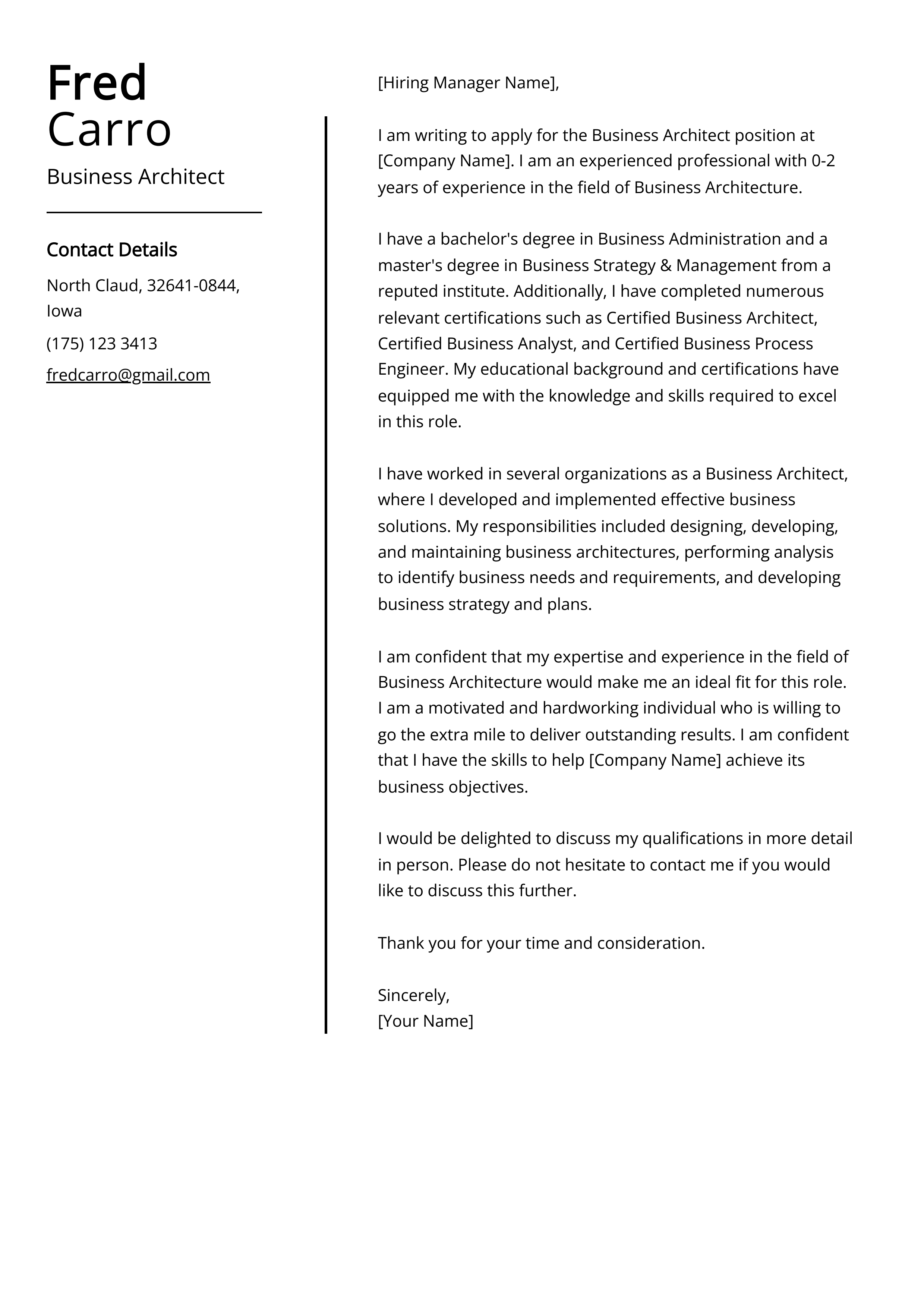The image depicts a professionally crafted cover letter addressed for a job application. Titled with the large text "Fred Kiro," who is a "Business Architect," the top left corner of the letter provides Fred's detailed contact information, including his address, city, state, zip code, phone number, and email. The letter begins with a polite salutation and states that Fred Kiro is applying for the position of Business Architect at a company. It highlights his substantial academic qualifications, including a Bachelor's degree in Business Administration and a Master's in Business Strategy and Management obtained from prestigious institutions. Fred also lists his numerous professional certifications such as Certified Business Architect, Certified Business Analyst, and Certified Business Process Engineer, emphasizing how these have poised him well for the role. Throughout the letter, Fred outlines his experience, specifying that he has zero to two years of practical experience in business architecture, which includes developing effective business solutions, designing architectures, performing business needs analysis, and formulating business strategies. The cover letter concludes with Fred expressing his enthusiasm and readiness to discuss his qualifications in more detail, asking for the opportunity to further detail his suitability for the role. The letter is courteously signed off with "Sincerely, your name placeholder."